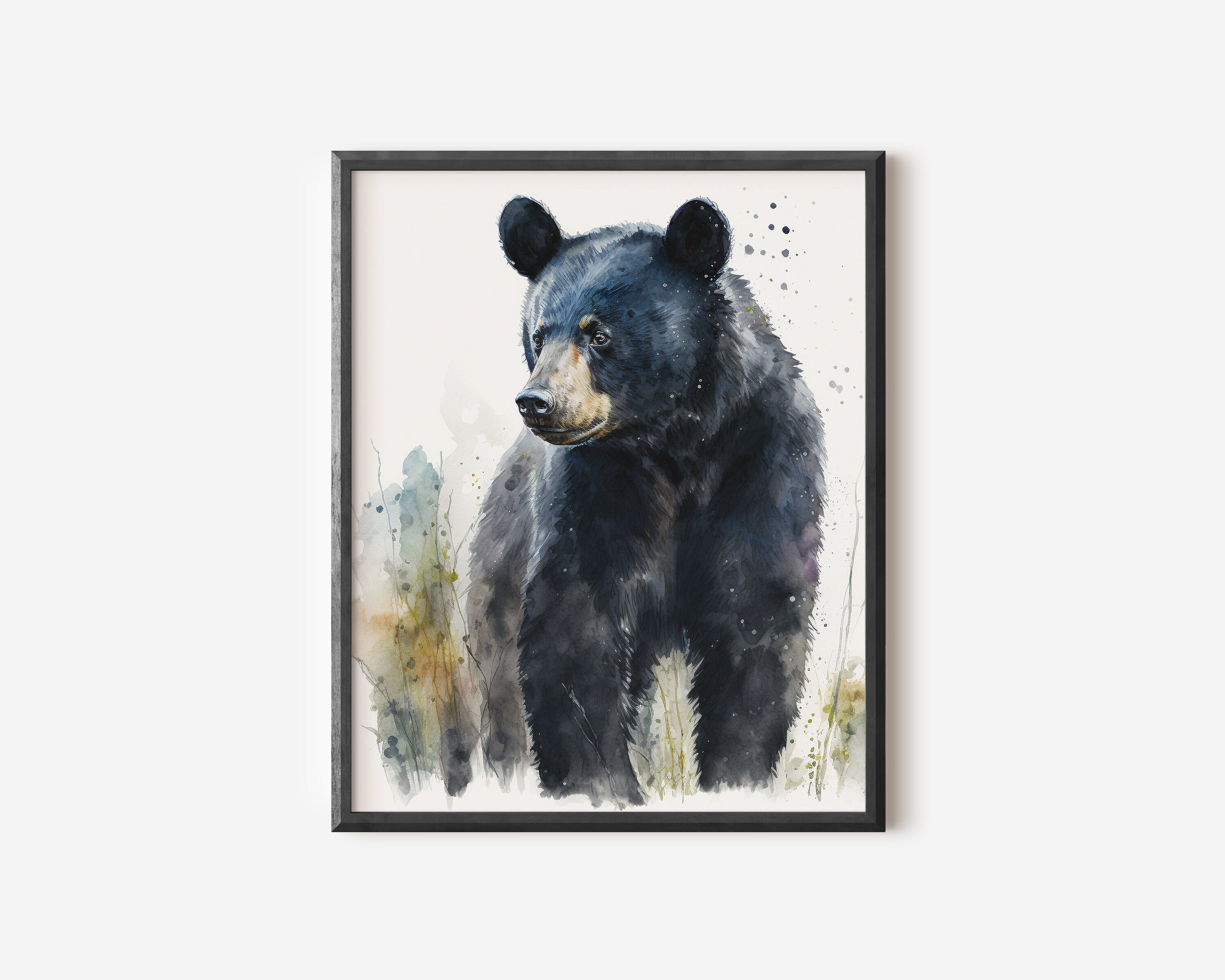This is a detailed artwork of a black bear, framed and prominently displayed against an off-white wall. The composition is set in a thin, black metal frame. The painting, which appears to be a combination of watercolor and colored pencil, showcases a large black bear, occupying most of the picture's space. The bear is positioned centrally, with its head turned slightly downward to the left. It has striking black eyes, a distinct light tan snout, and a serious expression on its face. 

The bear’s fur is a deep black, interspersed with shades of gray and white, especially toward its thick legs, which fade out toward the bottom of the artwork. Above the bear, the upper right corner features dynamic black and gray dots, giving the impression of the bear shaking off water. The background incorporates subtle hues of green, yellow, and blue, resembling bushes or foliage, adding a textured, natural feel to the scene. The artist has carefully detailed the bear’s environment with hints of grass and leaves in varying shades of gray, green, orange, and yellow, enhancing the overall wild and rugged atmosphere of the painting.